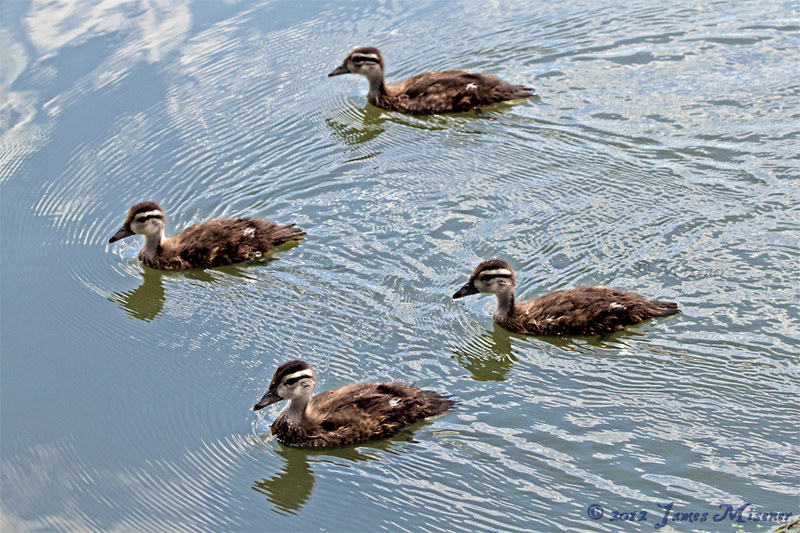This is a professional landscape photograph, signed "James Meisner, 2012" in blue font in the bottom right corner. The image captures an overhead view of a serene body of water, possibly a pond or lake, reflecting the blue sky and white clouds in the upper left corner. Four young mallard ducks, not yet fully mature, are swimming towards the left side of the frame, creating ripples that disturb the water's surface. The ducks, detailed with brown heads, white stripes alongside their eyes, tan faces, black beaks, and dark backs with a few white spots on their wings, are positioned with one in the lead, two flanking it, and one slightly trailing behind. The V-shaped wake following them adds dynamic movement to this tranquil nature scene.